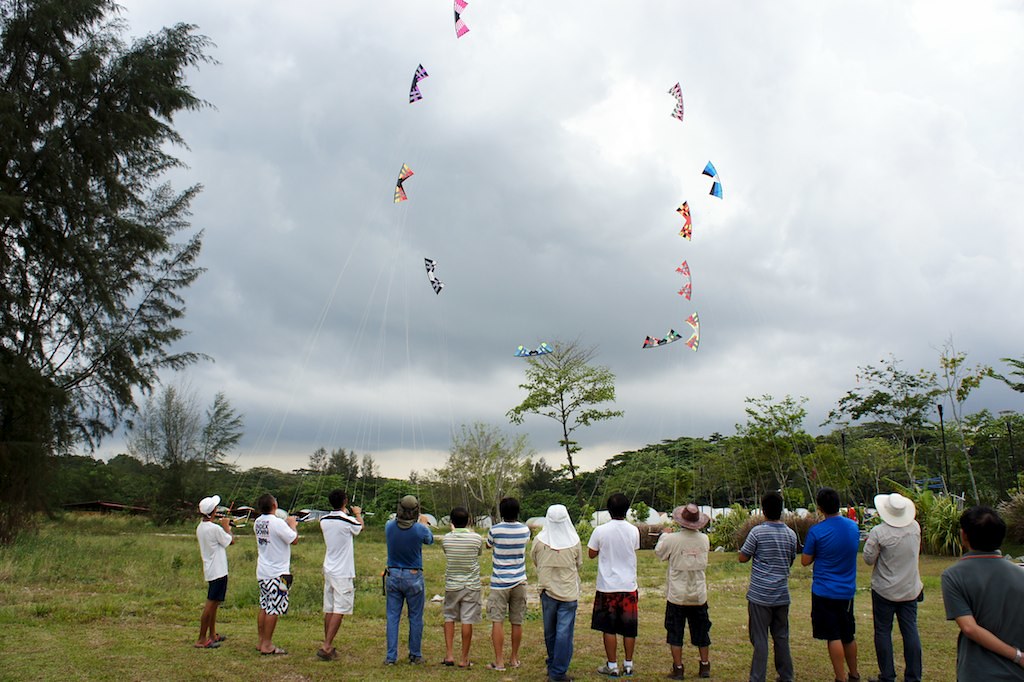The image captures a lively scene of approximately ten people standing in an open field, possibly a park, flying vibrantly colored kites against a cloudy gray sky. The grass beneath them varies between green and brown patches, and the background is adorned with an assortment of leafy trees and bushes in various shades of green, forming a picturesque horizon about a quarter of the way up from the bottom of the photograph.

Each person, casually dressed in shorts, jeans, t-shirts, and some with hats and sandals or tennis shoes, holds a unique kite aloft. The kites, not of traditional shape but featuring a curved outer part with two prominent "teeth," form an oval or circular pattern in the sky. The colorful array includes kites that are pink with white and blue accents, red with white and blue stripes, yellow with black, green, and orange hues, white with blue stripes on the wings, blue with white dots, a multicolored kite with black spots, yellow with blue stripes and red points, red and blue combinations, black with yellow and red patterns, as well as turquoise and dark blue, and white with red at the back.

The scene is harmonious yet dynamic, with the community coming together under a sky thick with clouds to partake in the joyous activity of kite flying, framed by the natural greenery of the park.